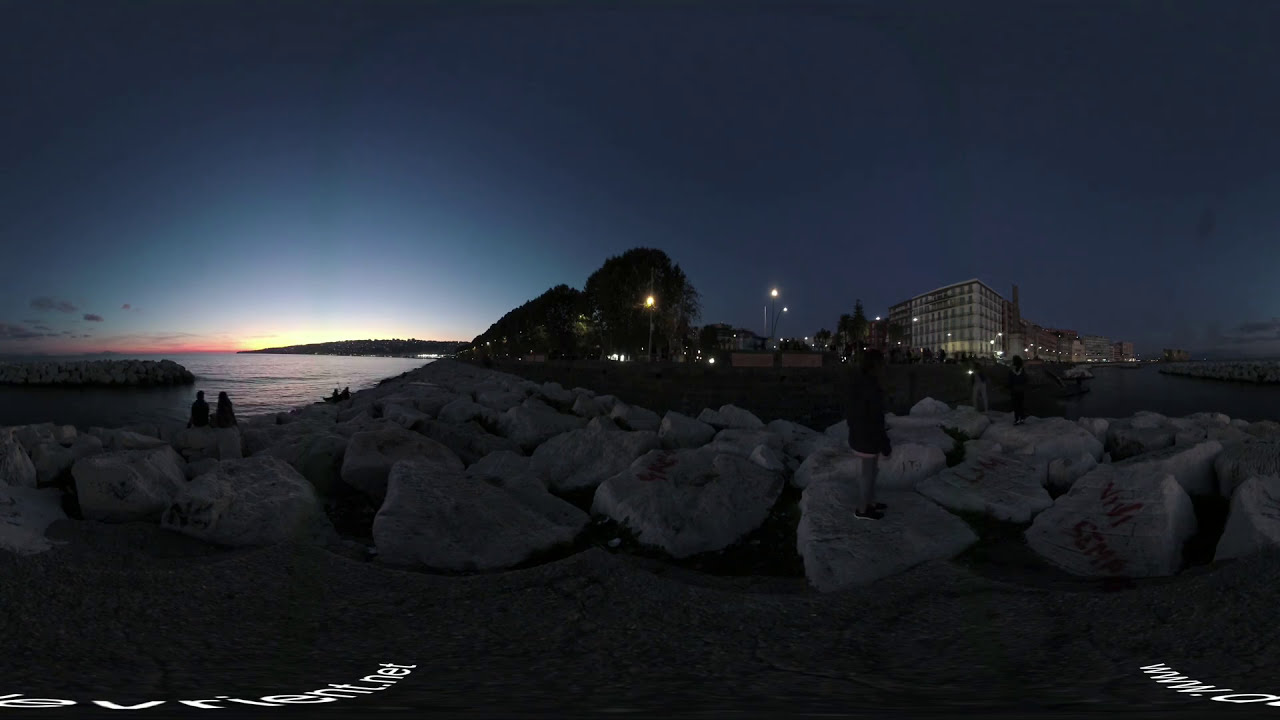This image captures a picturesque and romantic seaside scene taken just after sunset. The foreground is dominated by large gray and white rocks, some bearing indistinct dark red graffiti. To the left, a tranquil body of water, possibly a bay or part of the ocean, stretches out under a sky that transitions from deep blue to light pink and golden hues with subtle tints of red and yellow. Silhouettes of people populate the scene: a couple sits on the rocks near the water's edge, gazing at the horizon, while another person stands alone on a rock, also looking out over the water. To the right, the background includes trees and a large building, likely a hotel or urban development with street lights beginning to illuminate the area. The overall atmosphere is an enchanting blend of natural beauty and human presence, making for a captivating dusk setting.